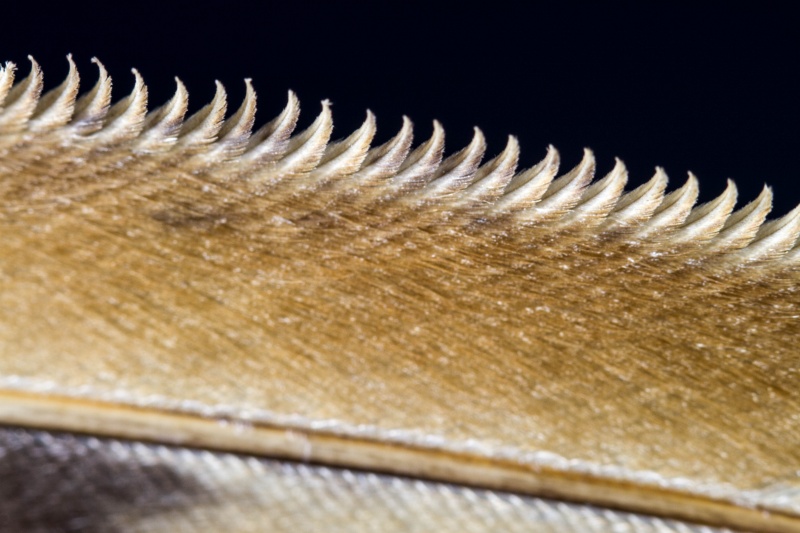This highly magnified image features several distinct layers of texture and color. At the top of the image, a row of small, white, fin-like shapes stretch horizontally across the frame. Beneath this, a section of light gray occupies the bottom, with a patch of darker gray in the bottom left corner. Directly above the gray portions, a tan and brown horizontal line creates a stark divide. Moving further up, a significant portion of the image is dominated by a light brown, scaly texture. Above the scaly section lies another row of roughly 20 small, white, fin-like shapes, closely aligned from left to right. Crowning the image, a solid black background extends across the top edge, providing a bold contrast to the detailed textures below.